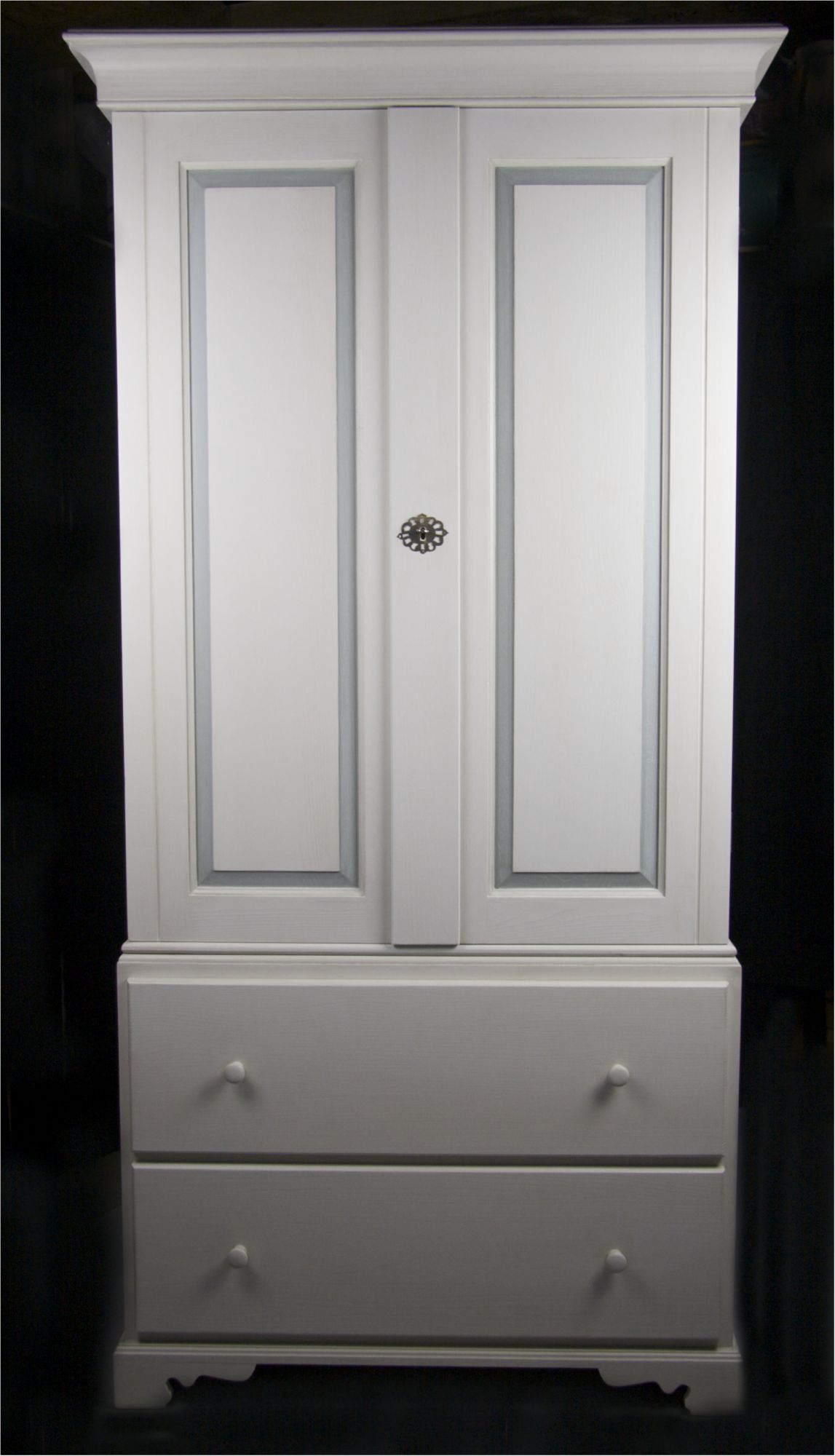This image features a tall white armoire against a dark black background, primarily occupying the majority of the frame. The well-lit top contrasts with the shadowy bottom. The armoire's upper section comprises two tall, closed cabinet doors. Each door is accented with a recessed, long rectangular panel trimmed in silver. In the center of where these doors meet, there is a decorative black floral-shaped keyhole with silver markings around it. Below the cabinet doors, the armoire has two pull-out drawers, each equipped with two round white wooden knobs, one on the left and one on the right side of each drawer. The entire piece appears to be made of wood, painted white, with a floral type knob where the doors meet and detailed silver trimming that adds elegance to its minimalist design.